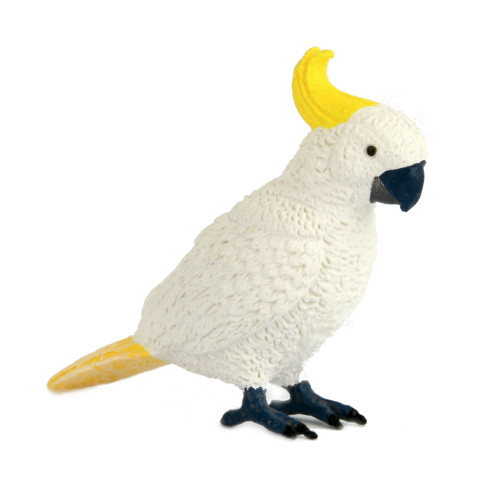The image depicts a detailed and intricately crafted model of a white parrot or macaw, made from a material resembling resin or possibly crocheted yarn. The parrot is positioned against a clean, white background, facing to the right. Its plumage is predominantly white, with a striking yellow crest extending from the back of its head in a wave-like formation, matching the bright yellow feathers of its tail. The bird has small, black eyes, and its beak is distinctive, with the upper part being black and the lower part a dark gray. The feet are a dark hue, appearing almost black, with each foot showcasing two toes with black toenails. This highly detailed and textured representation captures the essence of a parrot with a harmonious blend of white, yellow, black, and gray tones.